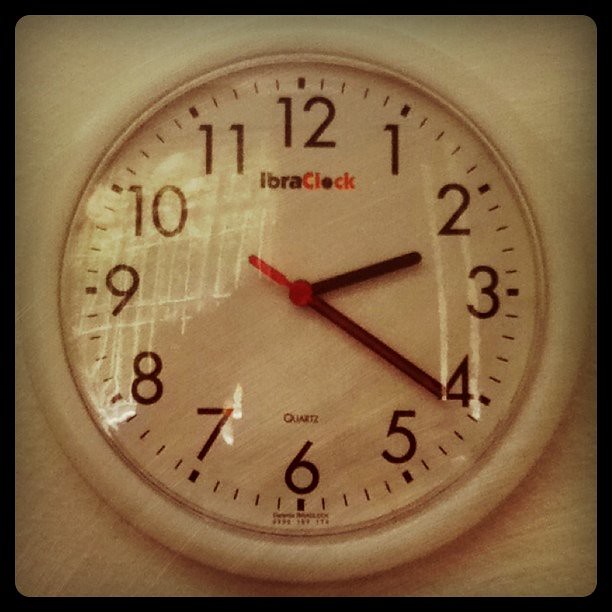This image presents a detailed depiction of a wall clock mounted against a grayish-white wall. The photo itself features a black border encasing a tan border. The round clock within these borders has a white plastic outer edge. The clock face, also white, is protected by a clear glass or plastic cover. The numerals 1 through 12 are marked in black around the clock, with black lines in between representing each minute.

The clock displays the time as 2:21 and 21 seconds. The hour and minute hands are black, while the second hand is red. Below the 12 o'clock position, the manufacturer's name “Ibroclock” is inscribed, with "IBRA" in black letters and "CL CK" in red, where the "O" is represented by a solid black circle. Above the 6 o'clock position, the word “Quartz” is written. The face, hands, and markings of the clock are all clearly visible and detailed, harmonized by the overall cream-colored background.